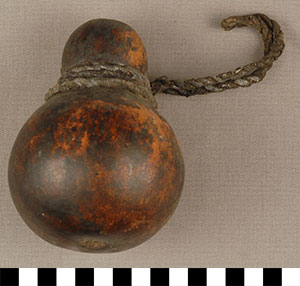The image depicts an old, wooden object shaped like a squash or gourd, featuring a weathered appearance with a mix of dark and light brown tones interspersed with patches of black. The surface of the object has a noticeable shine with two reflections of light visible near the bottom. A doubled-over rope, which appears to be quite old, is wrapped around the neck of the object at least twice, positioned towards the upper right side. The object rests on a dark gray background, possibly a table, although this is not entirely clear. The bottom edge of the image is lined with a strip of black and white checkered squares, adding a distinct border to the scene.